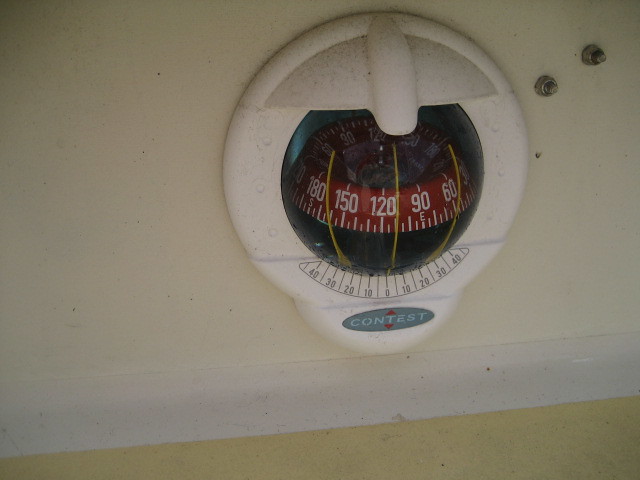This image features a detailed view of a white, likely retro thermostat, approximately 7 inches in height. At the center of the thermostat is a prominent red circular gauge with a 3D effect, recessed into the white outer frame. The circular gauge displays temperature measurements, starting from 180 degrees on the left, and progressing through intervals marked by smaller lines: 150, 120, 90, and finally 60 degrees. 

In the center of the gauge, there are three distinct yellow vertical lines. Below these lines, another set of numbers in gray begins at 40 on the left, decreasing through 30, 20, 10, and down to 0. On the right side, this gray scale ascends back from 0 up to 40, with intervals marked for 10, 20, and 30.

Beneath the central circular gauge, the brand name "Contest" is displayed. This branding sits within a blue circle framed by a tiny red arrow above and below it. Adding to the uniqueness of this thermostat, there are two small silver buttons located on the white wall to the upper right corner of the device. This combination of color, design, and intricate details contributes to an unusual and distinctive appearance, unlike any common thermostat typically encountered.